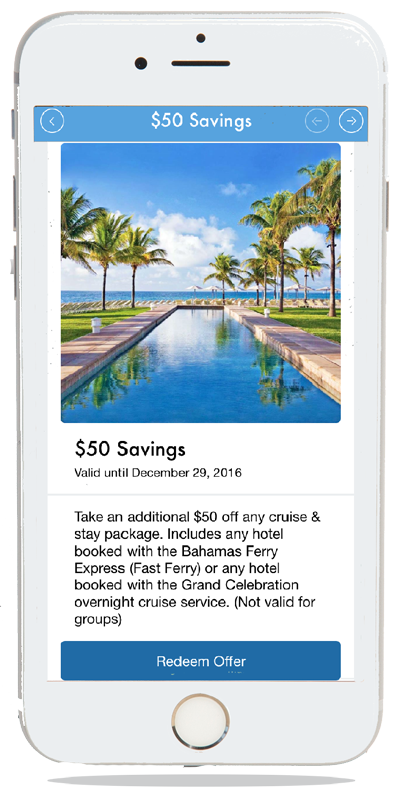The image depicts a white cell phone in a mock-up format, prominently displaying a promotional offer overlay for a travel package. The cell phone itself is fully visible, featuring a white trim and a white button centered at the bottom of the device. The main content of the screen is somewhat misaligned, as the promotional image does not fit perfectly within the display.

At the top of the screen, there's a horizontal bar with white text that reads "$50 savings." Below this, a vibrant photograph showcases a picturesque tropical beach scene. The foreground is dominated by clear blue water that forms a rectangular path flanked by wooden decking. On either side of the decking, green grass and tall palm trees add to the tropical ambiance. Further into the distance, the beach reveals umbrellas set against a stunning backdrop of the ocean, a bright blue sky, and fluffy white clouds.

Directly beneath the photograph, larger, dark text reiterates the "$50 savings" message. In smaller text just below this, the promotion is specified to be valid until December 29, 2016. A thin gray line then separates this information from further details of the offer.

The detailed text explains that an extra $50 discount is available on any cruise and stay package, which includes any hotel booked with the Bahamas Ferry Express (Fast Ferry) or the Grand Celebration Overnight Cruise Service, with the stipulation that the offer is not valid for group bookings. At the very bottom of the screen, a blue button stretches across the display, featuring the call to action "redeem offer" in bold white letters.